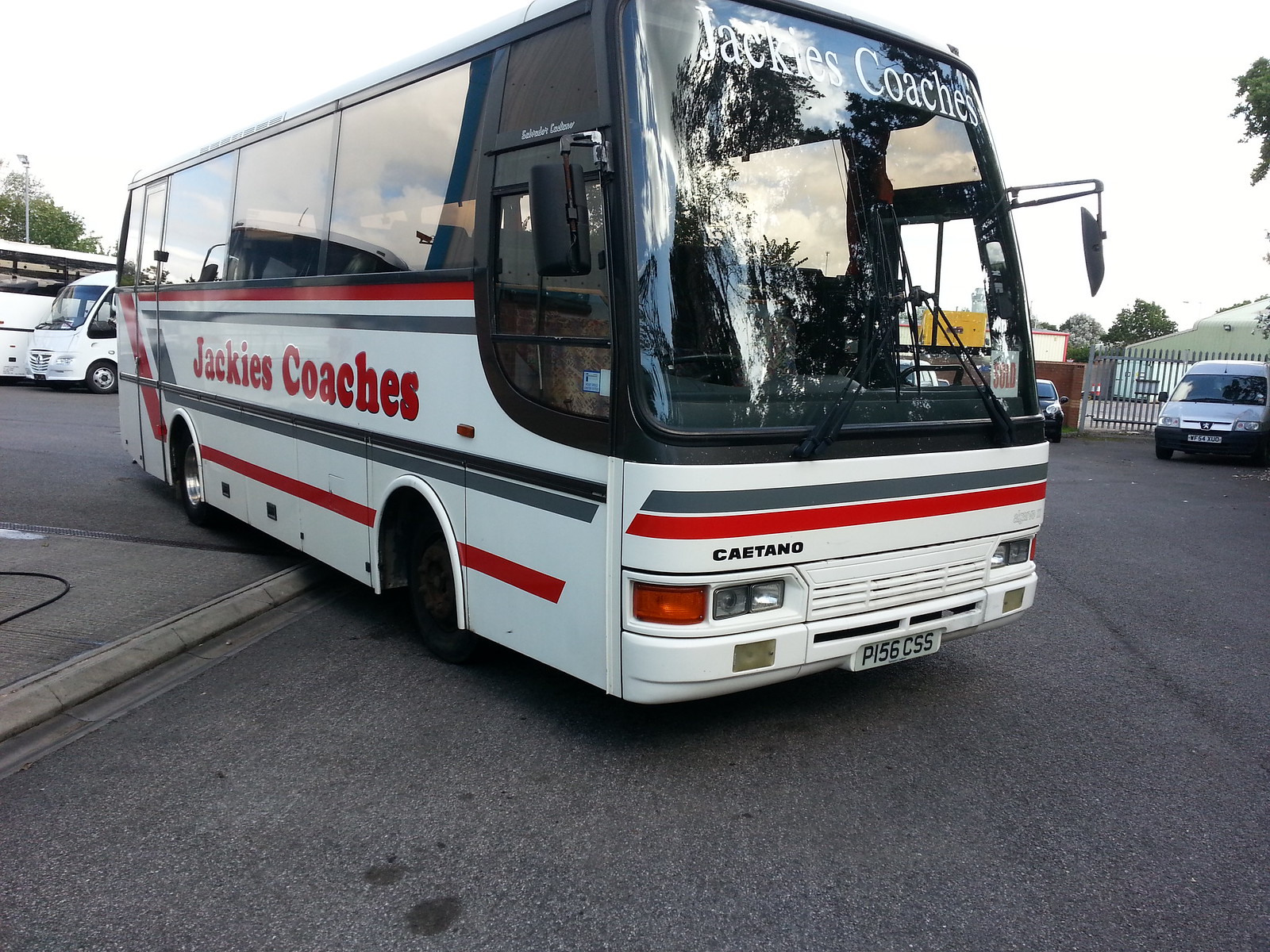The image features a large coach bus primarily painted white with distinctive red and blue stripes. Prominently displayed in red lettering on the side of the bus are the words "Jackie's Coaches." The same branding appears in white above the windshield. The bus is identified as a "Cayetano" model with the license plate "P156 CSS" visible on its front bumper. The coach appears to be parked, partially overlapping a sidewalk on a black asphalt road. Shadows cast by nearby trees obscure a clear view into the bus, but it seems unoccupied. A "SOLD" sign is displayed in the bottom right corner of the windshield, suggesting it might have recently been purchased. The background reveals other vehicles and coach buses parked, as well as some buildings behind a fence on the top right of the image, adding to the urban setting.